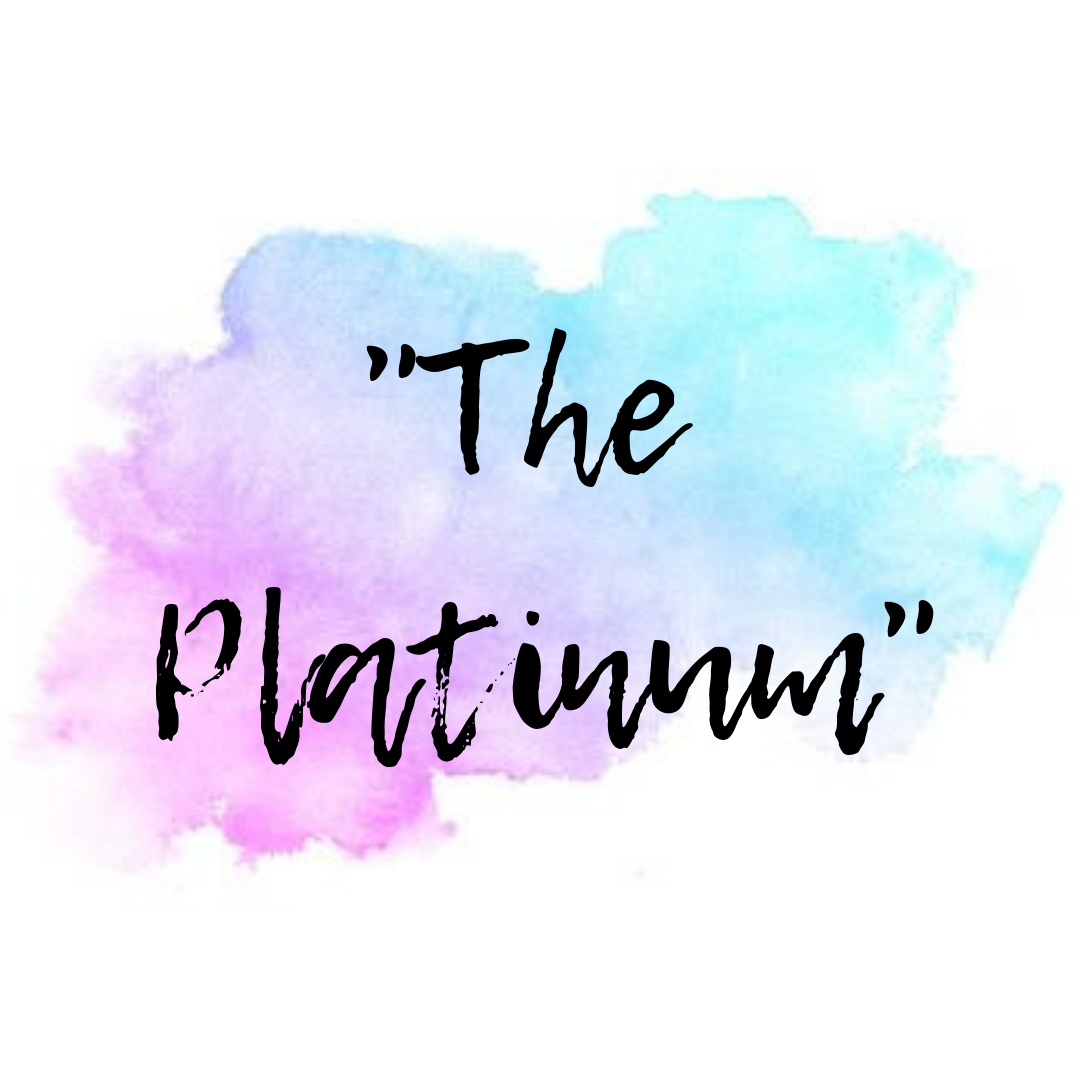The image features a predominantly white background with a centrally placed watercolor blob, resembling a cloud. This cloud-like shape transitions through an ombre effect, blending from a rich purple in the bottom left corner to a light teal in the upper right. At the center of this colorful gradient, there is a script-style handwritten black text that reads "The Platinum" in quotation marks. The font style is reminiscent of painted or handwritten cursive. The image subtly suggests visiting Beadaholique.com for all your beading supply needs, though this phrase isn't included in the pictured text.